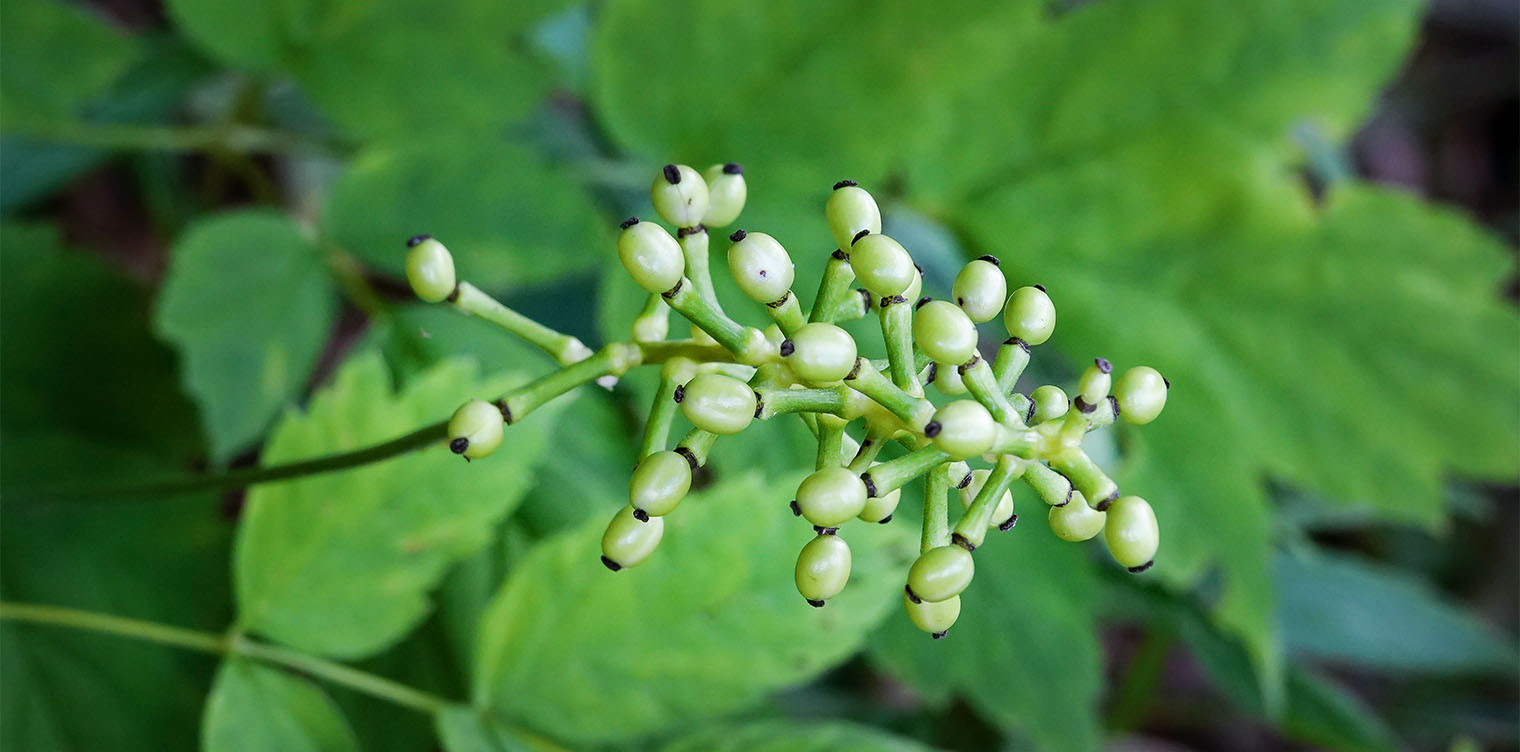In this close-up photograph, the focus is on an intricate part of a green plant, capturing the detailed structure of its pre-bloom buds. The main feature is a central, thin green stem, branching into multiple smaller stems each adorned with round, cylindrical buds. These buds are distinct with white round shapes culminating in tiny black dots at their tips. The composition highlights these bulbous buds pointing mostly to the sides, while the background is softly blurred, showcasing bright, vibrant green leaves that appear almost artificial due to their intense color. The photograph is angled such that the stem enters from the left-hand side, emphasizing the detailed textures and colors of the plant, set against a contrasting blurred backdrop.